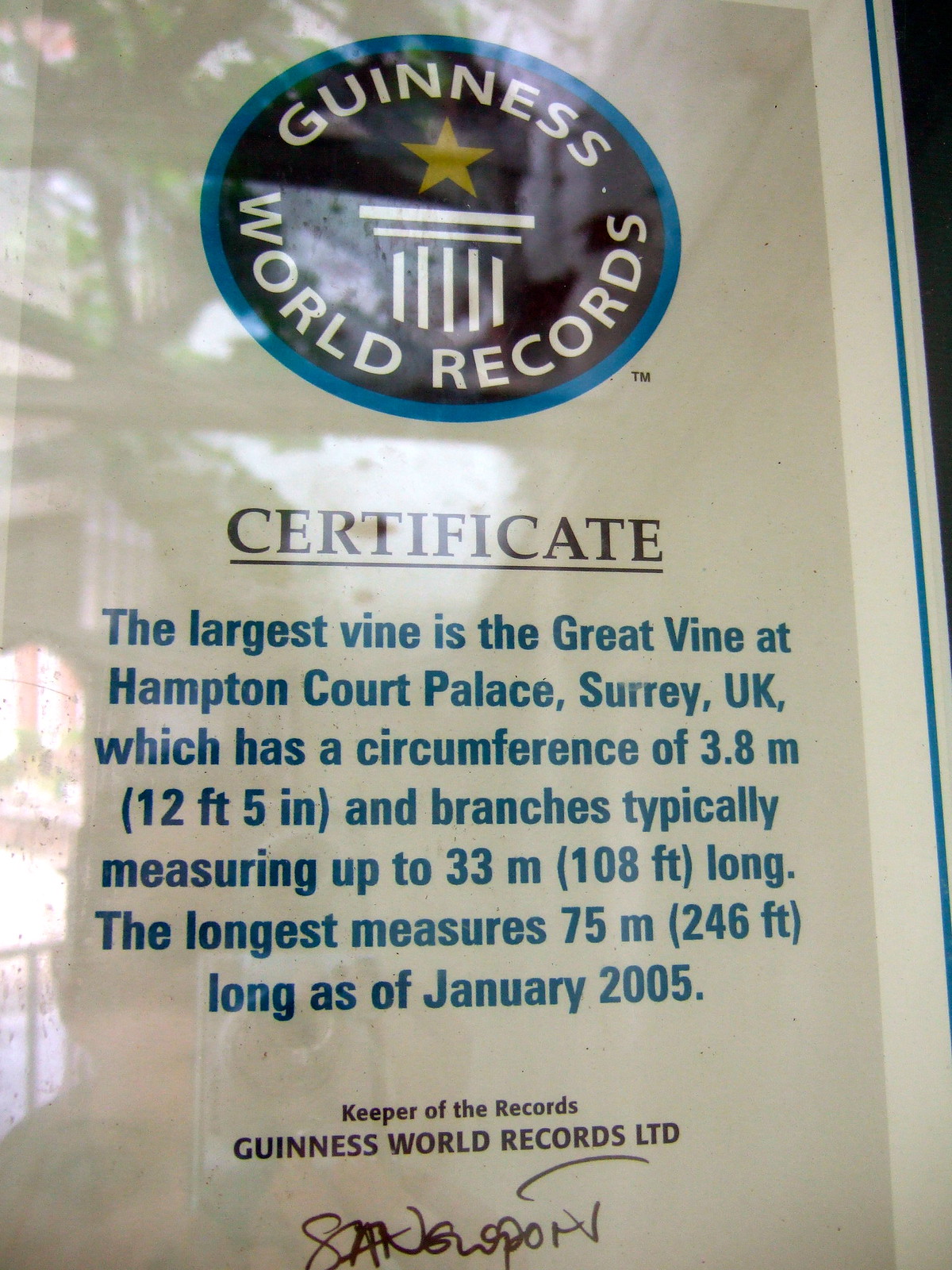The image showcases a framed Guinness World Records certificate displayed vertically under a reflective glass. At the top of the certificate is a blue circular emblem outlined in a lighter shade of blue. Within the circle, white curved text reads "Guinness" at the top and "World Records" at the bottom. Between these texts is a gold star over a pedestal with columns. Following the emblem is the word "Certificate," prominently written in capitalized, underlined dark blue letters. The main statement of the certificate reads: "The largest vine is the Great Vine at Hampton Court Palace, Surrey, UK, which has a circumference of 3.8 meters (12 feet 5 inches) and branches typically measuring up to 33 meters (108 feet) long. The longest measures 75 meters (246 feet) as of January 2005." Below the statement, in small black text, it states "Keeper of the Records, Guinness World Records LTD," followed by an illegible signature starting with 'S' and 'A.' The certificate is set against a white background, bordered by a white frame, with some light reflections visible on the glass surface.